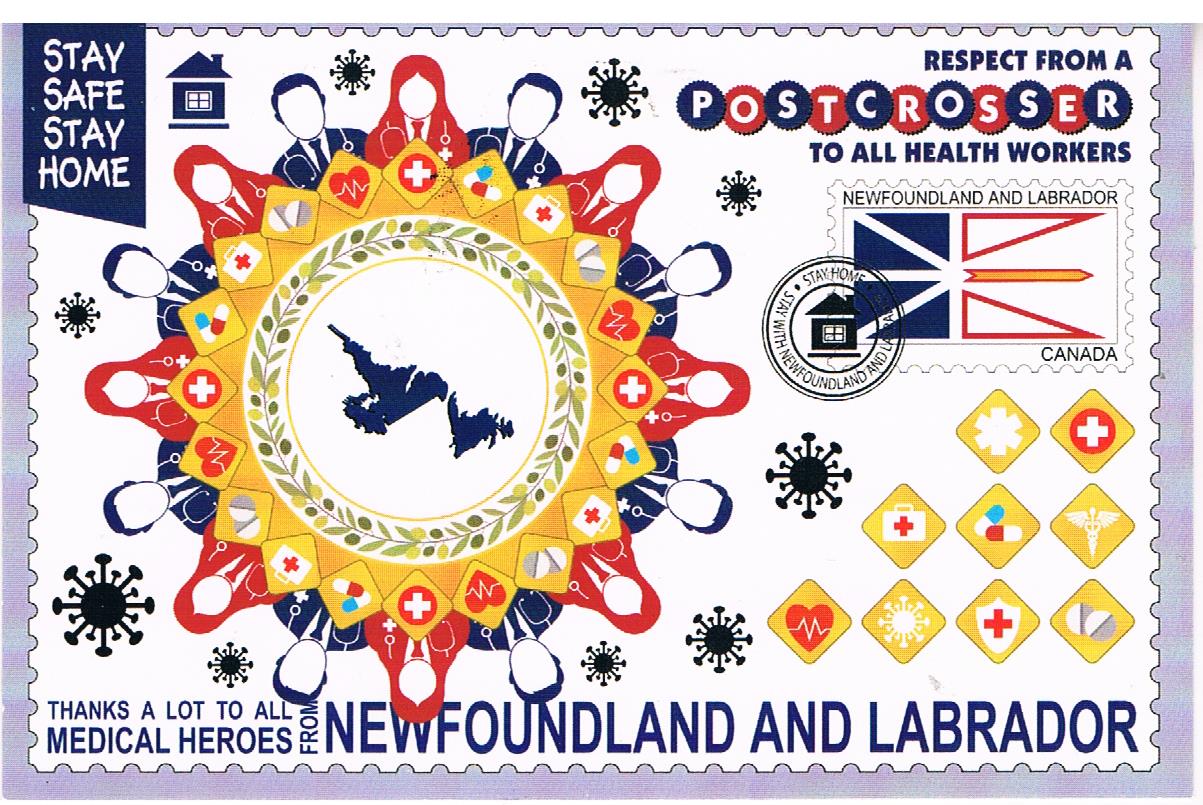This image is a brightly colored, highly detailed postcard dedicated to health workers. The postcard is bordered with a thin light blue line and features prominently the text "Stay safe, stay home" in white letters on a blue background at the top left corner, accompanied by an image of a house. Centrally, there is a large round yellow table-like surface edged with points and symbols, surrounded by illustrations of people from the chest up; men in blue and women in red, alternating around the circle. Below this centerpiece, the postcard reads "Thanks a lot to all medical heroes," with "from" positioned sideways, and "Newfoundland and Labrador" in larger text. 

On the top right, the text "Respect from a post crosser to all health workers" is displayed in blue and red circles with white letters, accompanied by a stamp featuring symbols and a postmark. Additional details include yellow diamonds filled with symbols, and the repeated phrase "stay safe, stay home." Various medical symbols such as pills, a cardiovascular health icon, a heart, a cross, and COVID-19 molecular structures decorate the postcard, emphasizing the message of appreciation and safety during the pandemic.